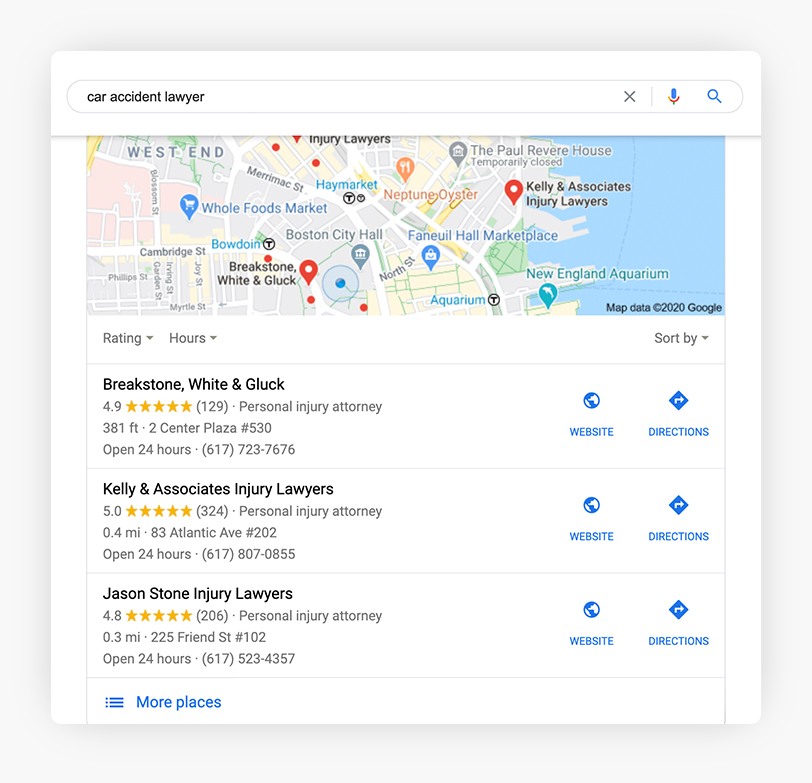A collage of various informational snippets reveals a vibrant background. In the top left corner, "Barnes" is mentioned as a car accident lawyer, accompanied by an icon resembling a microphone. The theme combines blue, matte, white, and glass elements. A section highlights Weston, characterized by a mix of blackstone, white, and black colors. Recognizable landmarks and businesses such as Whole Foods Market, Boston City Hall, Newell Health Marketplace, and New England Aquarium add community flavor. 

A prominent mention of "Kelly and Associates, Injury Lawyers" showcases details of their services, illustrated with a crisp blue website link and a "Directions" option. The Palo Verde House and vibrant clothing appear alongside a note about Neptune Oyster, illustrated near an ocean on the right. Ratings and operational information are peppered throughout the image, such as:

- Kelly and Associates, Injury Lawyers: Rated 5 stars by 324 reviewers, located 0.4 miles away at 83 Atlantic Avenue, Suite 202. They operate 24 hours and can be contacted at 617-807-7555.
- Deuce and Stone, Injury Lawyers: Rated 4.8 stars by 206 reviewers, located 0.3 miles away at 225 Friend Street, Suite 102. They also operate 24 hours and can be contacted at 617-523-4357.
- An additional listing with 4.9 stars from 1 to 9 reviewers, located at 3132 Center Plaza, Suite 530, with 24-hour availability, reachable at 617-723-7676.

The image also indicates the presence of more places, accessible online.